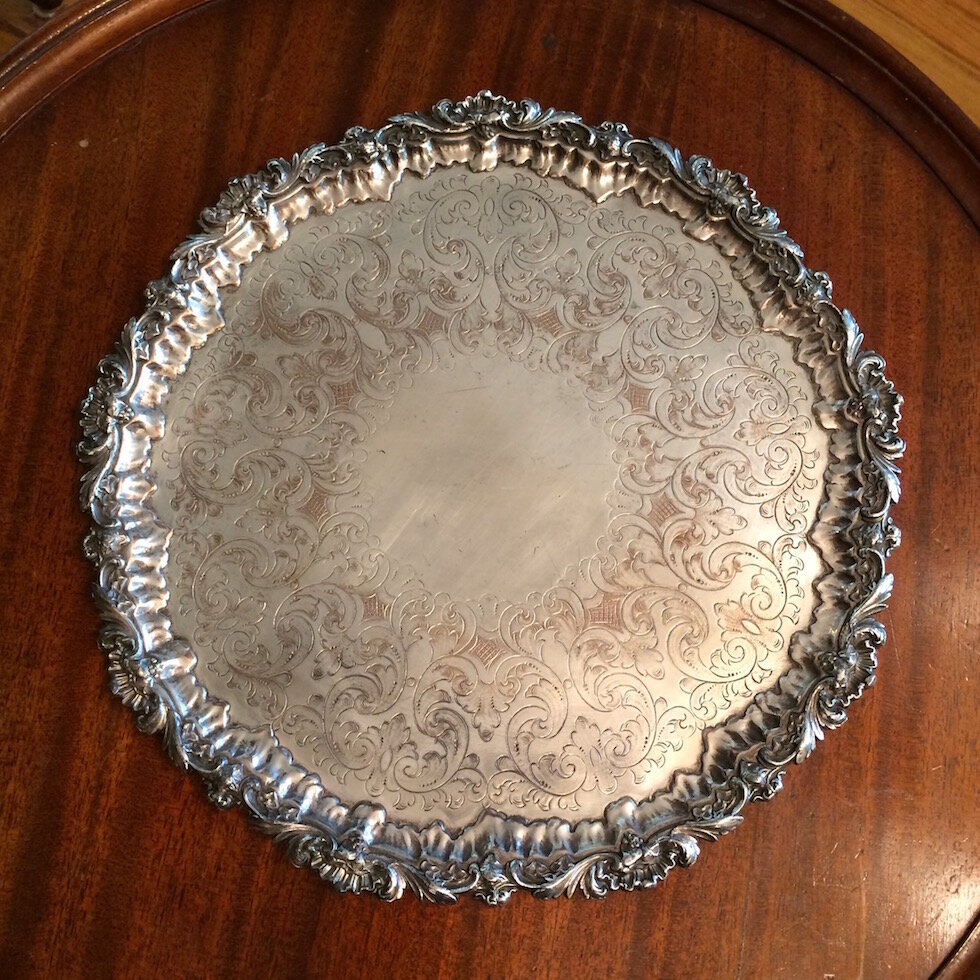This image, taken from directly above, captures a finely crafted antique scene. At the center, an ornate silver serving platter dominates the visual field, placed on a dark-stained, curved-edged, circular wooden table, suggesting antique origins. The platter itself showcases a spectacularly intricate border, adorned with an elevated, ornate floral vine design that rises above the plate's edge and transitions into a gold hue, possibly due to sunlight reflection. The inner border of the platter continues with an elaborate floral pattern featuring 'S' and backward 'S' shapes, along with intricate etchings and cross-hatching detail. This intricate design spans the outer surface but leaves the central section of the platter plain, providing a striking contrast. The silver displays varying shades, with the border having a darker, perhaps tarnished, silver tone with hints of bronze and brown, while the inner section remains a pale silver. The overall setting and intricate detailing highlight the craftsmanship and timeless elegance of the antique silver platter.